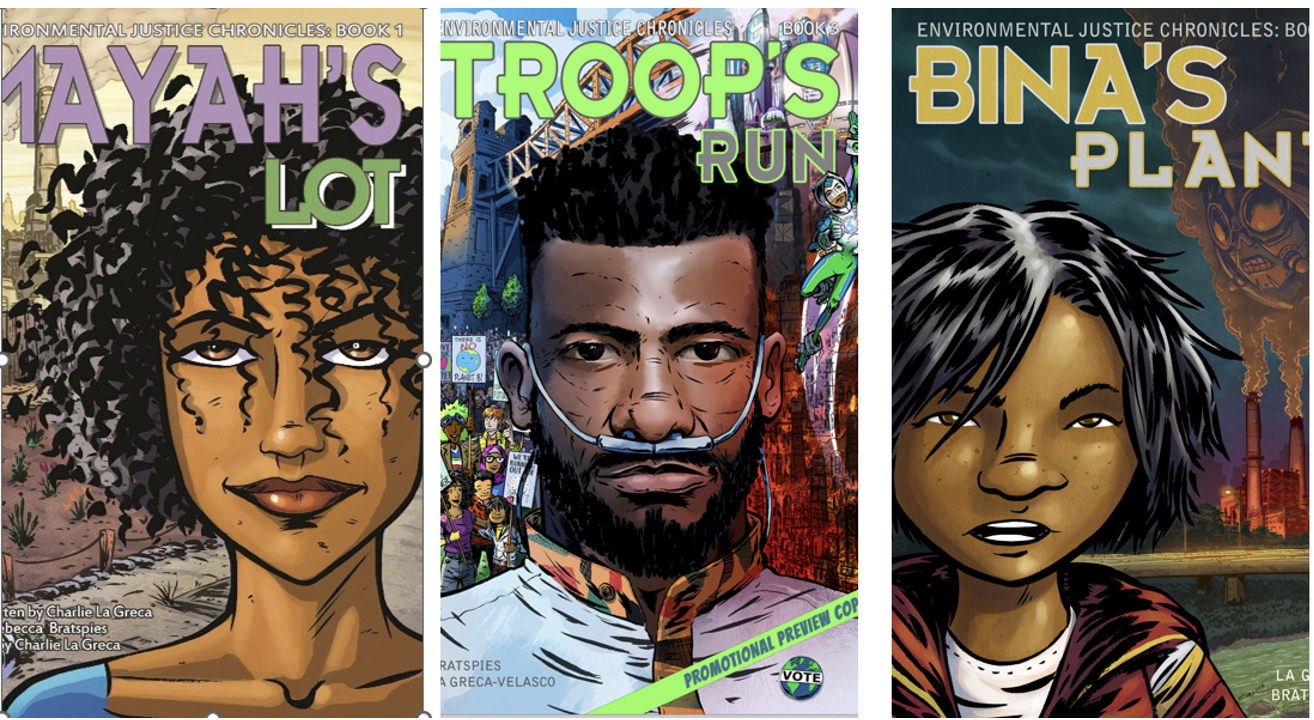The image showcases three color illustrations arranged in a row, each acting as a cover for comic publications. These covers are all in portrait orientation and depict a cartoon character from the head to mid-shoulders, each looking at the viewer.

On the leftmost cover, a young African-American woman with brown skin and long curly black hair is shown, looking up with a serious expression. She is wearing a blue shirt. The cover features the text "Iron Mental Justice Chronicles Book 1" in lavender and green, along with the title "Aya's Lot."

The center cover portrays an African-American man with a serious expression, wearing a white shirt. He is equipped with an oxygen tube in his nose. The text at the top reads "Iron Mental Justice Chronicles Book 3" in lime green and gray, with the title "Troops Run."

The rightmost cover features a young dark-skinned woman with black spiky hair, dressed in a dark red jacket. Behind her, a building is on fire. The text at the top is "Environmental Justice Chronicles" in small white letters, with the title "Bina's Plan" in gold and cream.

Each cover shares a similar comic book style with vibrant colors and consistent typography, emphasizing various justice themes and narratives.